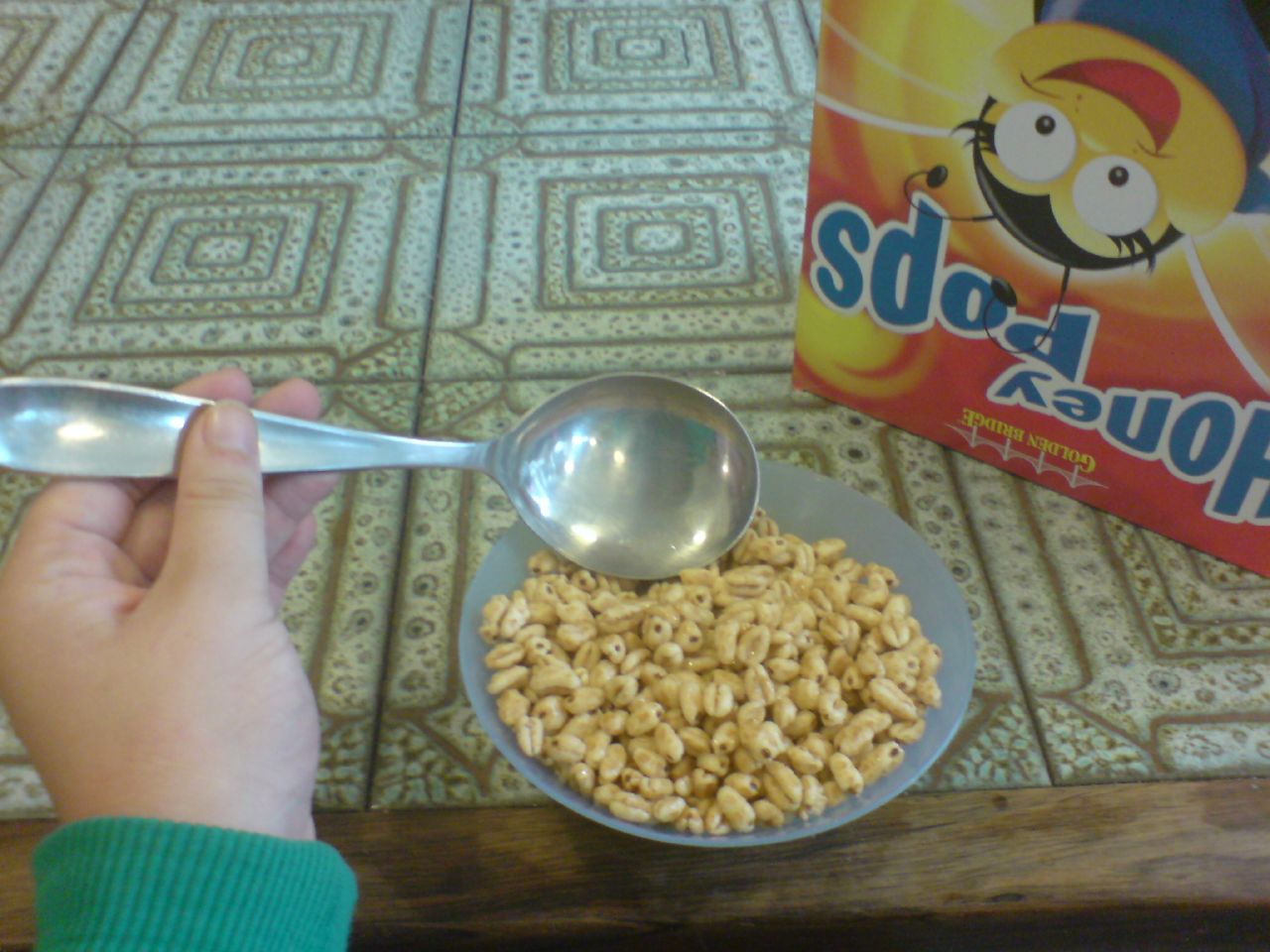This color photograph captures a detailed scene of someone about to eat a bowl of cereal. Central to the image is a small blue bowl, filled with puffed oat-shaped cereal identified as Honey Pops, as indicated by the upside-down cereal box to the right. The box is red and prominently features a cartoon bee, clearly readable despite its orientation. A left hand, possibly that of a small child due to its size, emerges from the bottom left, clad in a teal aqua blue sleeve. The hand holds a stainless steel spoon that delicately touches the cereal, suggesting the meal is about to begin. The bowl rests on a table adorned with a geometric or mosaic tile design, predominantly featuring shades of green, light green, off-white, and delicate gold, adding an elegant backdrop to the simple breakfast scene.